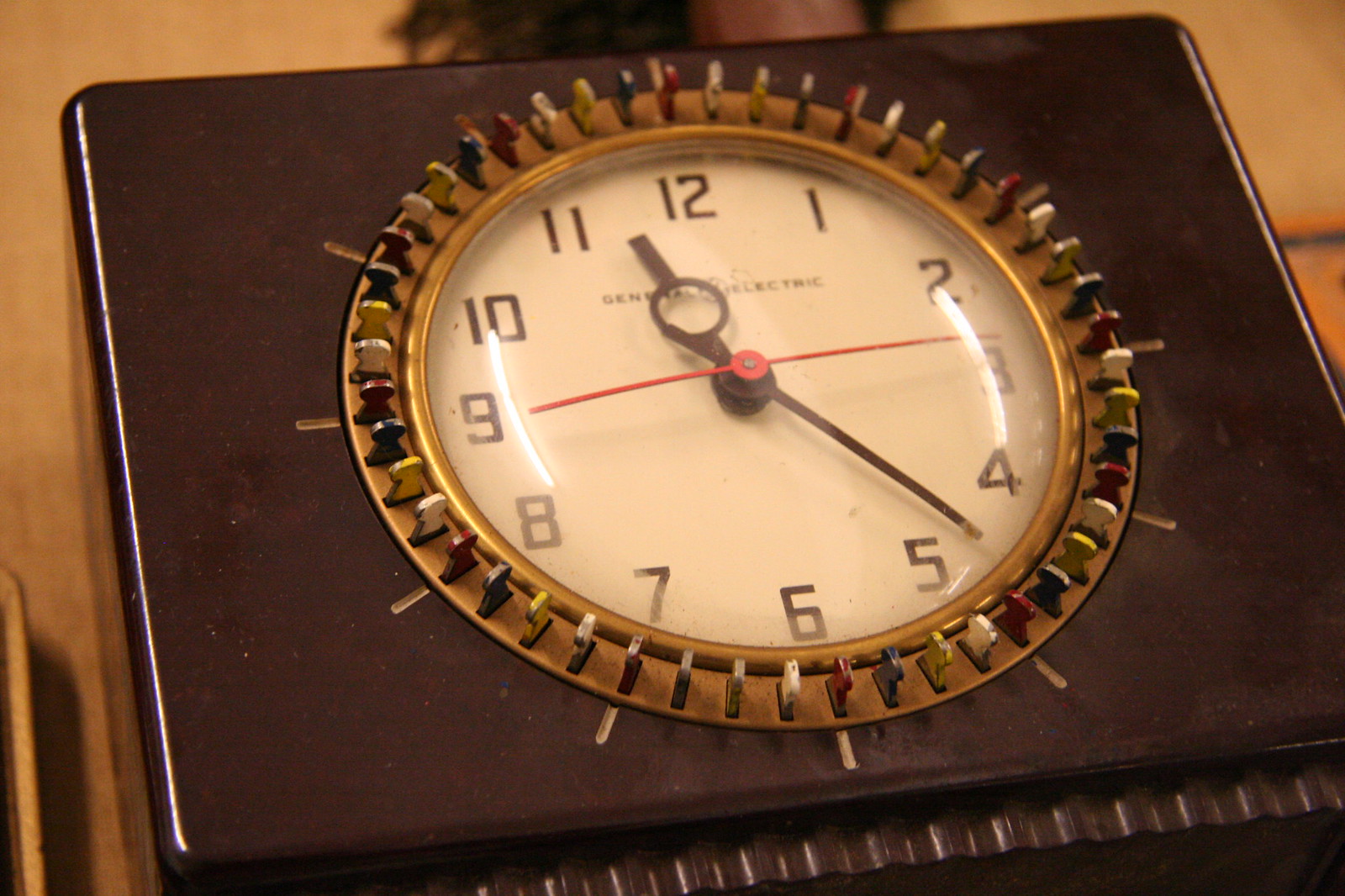This is a color photograph of a clock set into a dark brown rectangular wooden device. The clock has a cream face with black numbers from 1 to 12, black hands for the hours and minutes, and a red second hand indicating the time at 11:23. Surrounding the face of the clock is a gold rim from which various small metal pieces or keys jut out. These keys are in different colors, including yellow, white, dark green, and red, arranged in a repetitive sequence around the clock. The clock appears to display some brand writing, potentially "General Electric," although it is somewhat difficult to read. The glass over the clock face reflects light around the numbers 2, 3, 8, and 9, adding a glint to the image. Behind the clock, a blurry tan background provides contrast to the detailed clock and its colorful adornments.